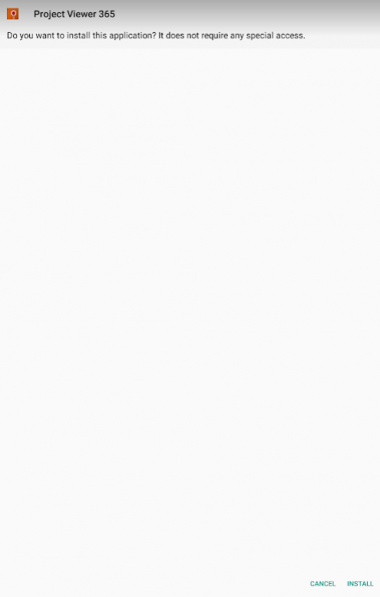The image captures a cropped screenshot of the Project Viewer 365 installation page. The screenshot, seemingly taken on a mobile device, is rectangular and elongated. At the top, a gradient gray-colored header transitions from dark at the top to light at the bottom. In the top-left corner, "Project Viewer 365" is displayed in bold black print. Just below this, a prompt in small black letters asks, "Do you want to install this application? It does not require any special access." The remainder of the page is predominantly white, with nothing else on it. At the bottom right corner of the screenshot, options to "Cancel" and "Install" are presented in small blue letters. The simplicity of the page accentuates the basic installation prompt for the Project Viewer 365 application.